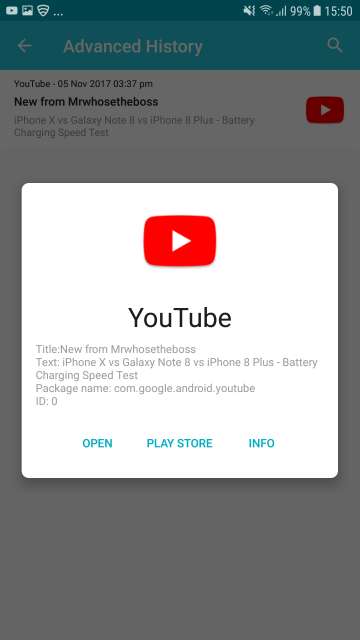The image displays a cluttered smartphone interface with several embedded elements:

- **Top Left Corner**: The YouTube app icon is prominently shown.
- **Main Display**: 
  - A partially visible image.
  - An array of notifications.
  - Signal strength and Wi-Fi indicators show full connectivity with a 99% battery level.
  - The time displayed is 15:50 (3:50 PM).
  - The screen appears unfocused and slightly obscured.
  - Several app icons and labels are visible, including a metronome clock.
  - A YouTube notification indicates a new video from "MrWhosTheBot" titled "iPhone X vs Galaxy Note 8 vs iPhone 8 Plus - Battery Charging Speed Test", uploaded on November 5, 2017, at 3:37 PM.
- **Additional Elements**:
  - A red square possibly highlighting a specific notification or app.
  - Mentions of "blue" associated with the Google Play Store.
  - An overall blue theme hints at the predominant color scheme.
  - The screen's grey border features rounded edges.
  - Some text is grainy, indicating low resolution or a poorly captured screenshot.

This detailed description attempts to encapsulate the state of a smartphone's screen filled with various icons, notifications, and an overarching blue color scheme.